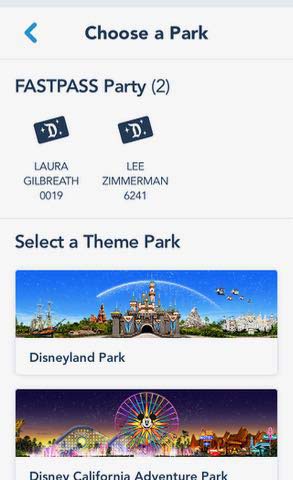The image features a sophisticated layout on a shaded gray background. At the top center, the text "Choose a Park" appears in black, accompanied by a small blue arrow pointing to the left. Below this, the text "Fast Pass Party (2)" is displayed in black. Underneath, two identical navy blue boxes with a white 'D' and three stars are included.

The first box is labeled "Laura Gilbreth, 0019" and the second "Lee Zimmerman, 6241." A fine gray line separates these names from the next section.

Heading the next section is "Select a Theme Park," followed by two options: "Disneyland Park" and "Disney California Adventure Park." 

For Disneyland Park, there is an illustrated depiction: the backdrop is a clear blue sky, showcasing the iconic castle. Flanking the castle, some rides are visible on both the left and right sides, providing a complete view of the park's entrance.

Below this, another image represents Disney California Adventure Park during nighttime. The sky is an enchanting mix of purple, yellow, and orange shades. A roller coaster is outlined on the left, while a Ferris wheel with Mickey Mouse at its center takes the middle of the scene. The Ferris wheel's spokes are vibrantly colored in purple, blue, and pink. The park is lit up with various lights, highlighting buildings, stands, and rides on the right.

The bottom image depicting Disney California Adventure Park is cut off just below its title.